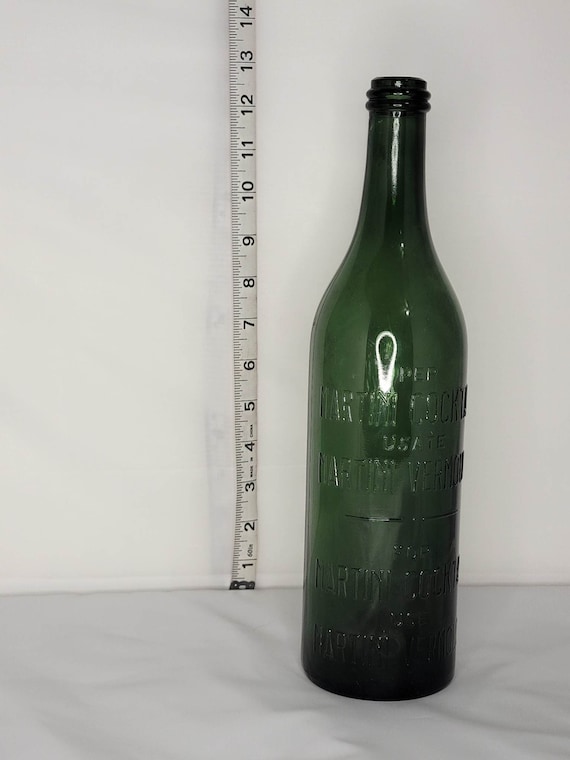The image features a vintage, dark green glass bottle, likely used for wine or soda, positioned on a slightly wrinkled white surface against a white wall. The bottle, seen fully from top to bottom and viewed from the side, has three rows of indistinct writing engraved into the glass. A white tape measure with black numbering is mounted on the wall directly behind the bottle, spanning from 1 inch to 14 inches. The tape measure indicates that the bottle stands approximately 13 inches tall. The predominant colors in the image are white, black, gray, and green, creating a monochromatic and somewhat nostalgic atmosphere.